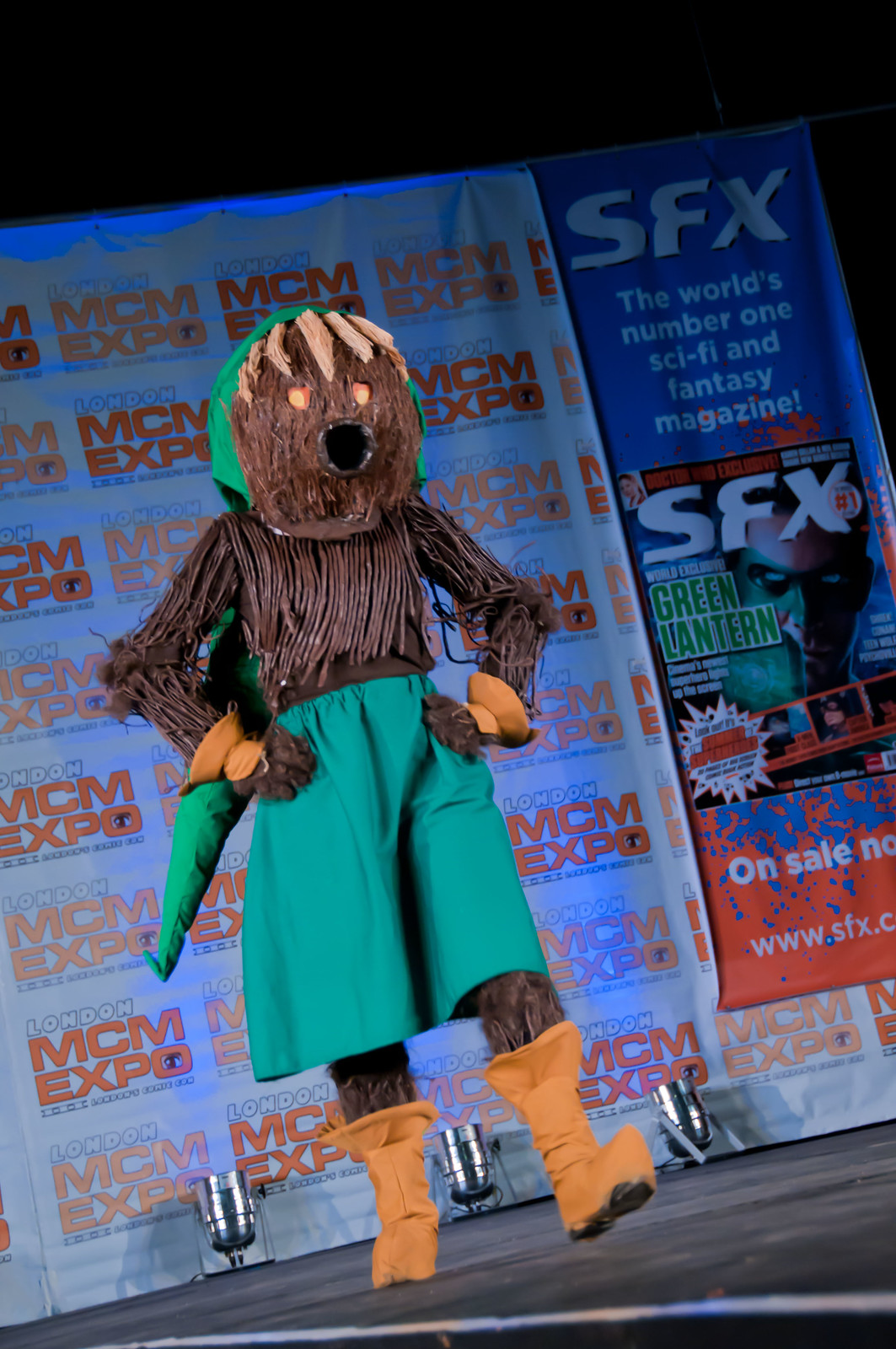The image, a color photograph in portrait orientation, depicts a character in an elaborate costume walking across a dark stage. The character sports a large, round brown mask adorned with two orange circles at the top, resembling eyes, and a black tube-like hole for a mouth, giving it an eerie, almost ominous expression. Straw hair cascades from the mask like bangs, partially covered by a green scarf wrapped around the head. The upper body is clad in a bodice made of strands of dark brown straw, paired with beige, fanned-out wristbands or gloves over brown gloves, which rest on its hips. The lower half features vibrant green shorts resembling culottes, fanning out similarly to a skirt, and is completed with beige boots. The background reveals a wall banner displaying the logo for the London MCM Expo, with "London's Comic Con" and "SFX: The World's Number One Sci-Fi and Fantasy Magazine" prominent in clear and orange typography. The character, reminiscent of a forest spirit or an anthropomorphic tree, evokes a fantastical and slightly sinister presence, possibly participating in a performance or cosplay event at the expo.